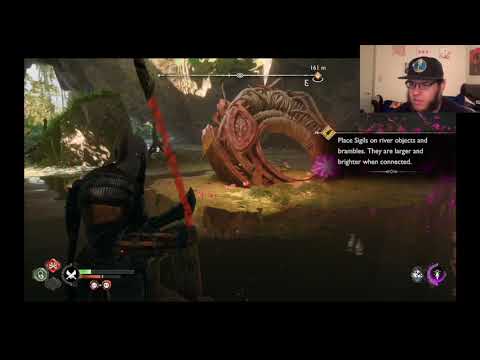The image is a screenshot from a video game stream, bordered by black widescreen bars on the top, bottom, and thinner vertical bars on the sides. In the upper right-hand corner, an inset shows the streamer, a man with lighter skin who is deeply focused on the game, his face framed by dense, bushy sideburns and adorned with black rectangular glasses. He wears a black baseball cap with a blue circular design and a black t-shirt. Below his image, text reads, "Place sigils over the objects and breakables. They are larger and brighter when connected."

The main game image features a forest-like setting with green land and trees. On the left side stands a warrior, clad in black shoulder pads, leather gloves, and a gray metal helmet. The warrior holds a red beam of light above the hilt, resembling a sword or staff. In the center of the scene is a large, circular stone object embedded in the ground, adorned with leaf-like patterns. Other unidentified objects, possibly animal-like figures, are scattered in the background, with a reddish-tan shape and a blackish item visible on the left and right.